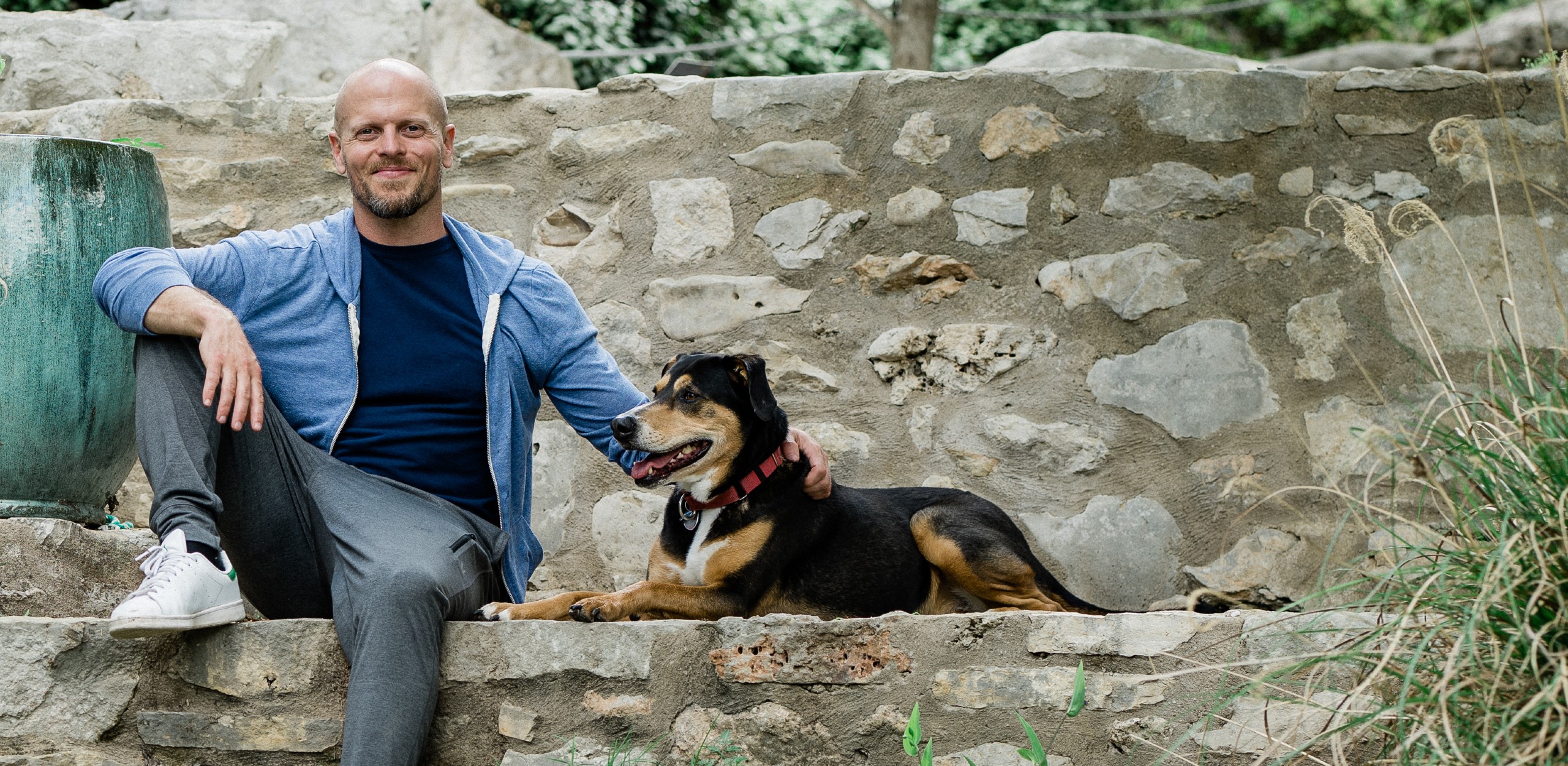This is a detailed photograph in a horizontal rectangle of a bald white man with a short brown beard, smiling, and sitting on a stone bench outdoors. He's positioned on the left side of the image, dressed in a light blue jacket over a dark blue T-shirt and gray sweatpants. His left leg is draped over the wall while his right leg is bent, with his foot resting on the ledge and adorned with a white tennis shoe. His right arm rests on his right knee, and his left arm is extended, petting his medium-sized black and brown dog with a red collar sitting to his right. The dog features more black on its back, with brown on its legs, belly, face, and a bit of white on its chest, and it is facing slightly forward with its mouth open. Behind the man is a stone wall and above it, some rock and greenery. To the far left, part of a green object resembling a vase or container is visible. The bottom right-hand corner of the image shows some grassy weeds emerging, enhancing the natural outdoor setting.